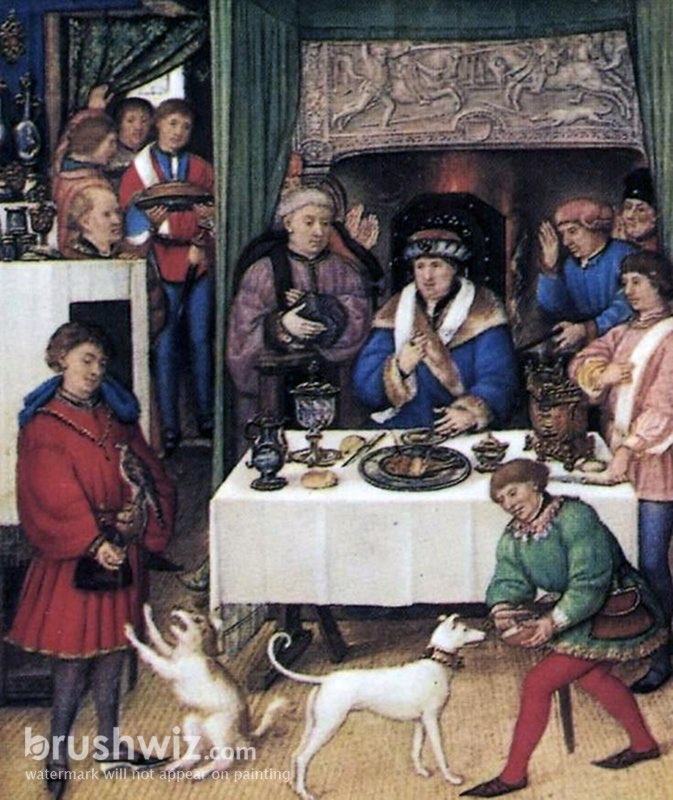The painting captures a vivid scene from the 16th-17th century, showcasing an ornate gathering with rich, historical detail. Central to the artwork is a man seated on a majestic black throne-like chair adorned with blue and brown fur-trimmed robes and a brown hat with white trimmings. He is located slightly to the right of the center, seated at a table laden with food and drink, including a plate and a goblet. Around him are several servants and attendants, with two on his left side and one on his right, who appear to be bringing him various items.

To the left side of the painting, there is a figure in red robes holding a bird, adding a touch of intrigue and exoticism. In the bottom foreground, a smaller person dressed in a green top and red pants is seen giving a treat to a white dog, while a white cat roams beside them. Nearby, another servant in red is also engaging with the dog. Further left, near the edge of the painting, kitchen staff bustle about, with two members emerging from a doorway carrying plates of food.

The backdrop features a tapestry or relief in shades of brown, adding to the medieval atmosphere. The bottom left-hand corner of the image bears a watermark that reads "brushwiz.com" alongside the note "watermark will not appear on painting," ensuring the viewer that the actual artwork remains undisturbed.